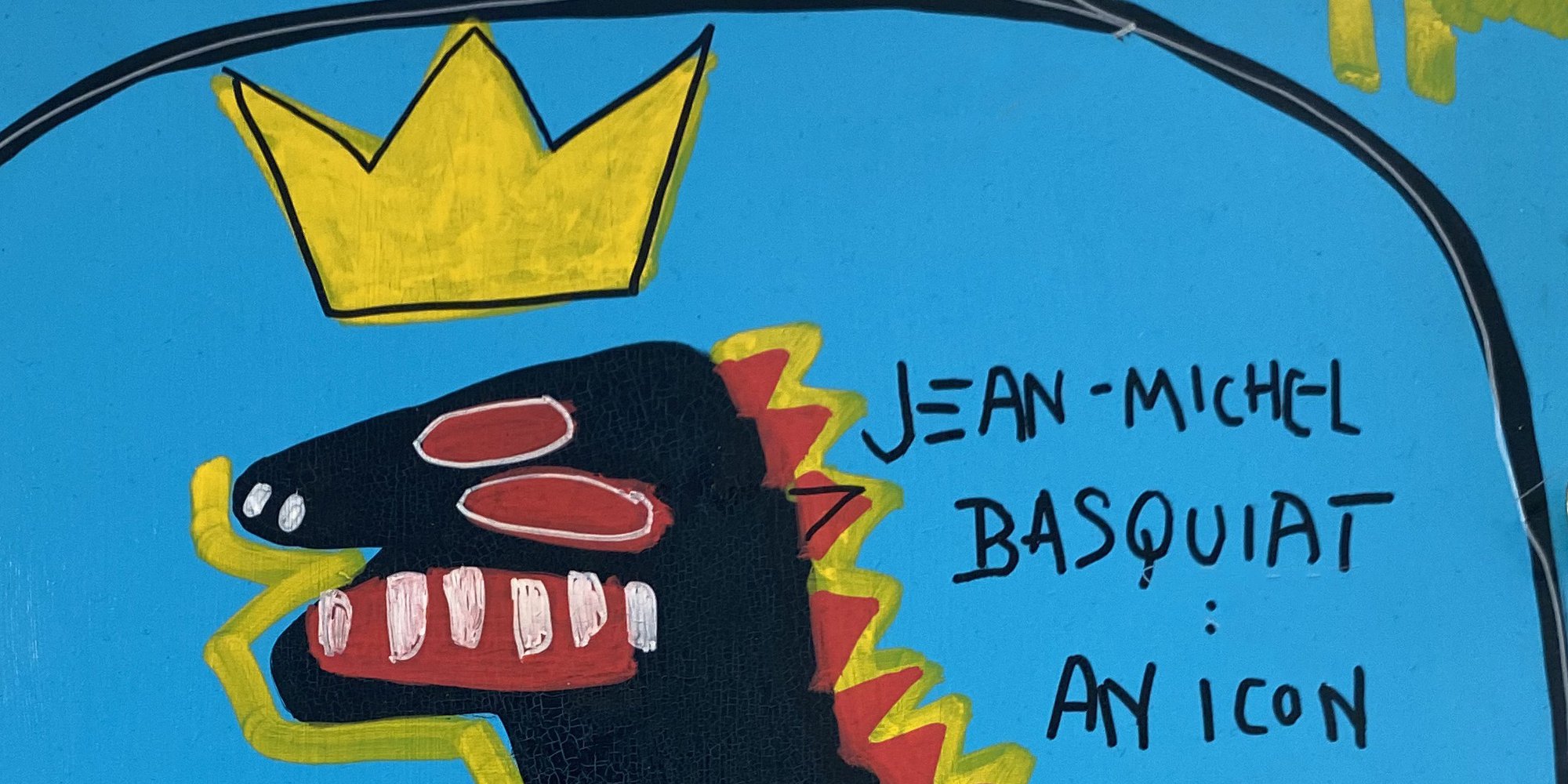This artwork is an old print attributed to Jean-Michel Basquiat, featuring a black dragon characterized by its comic book style, consistent with the artist's other works. The dragon, prominently positioned slightly left of center, has vivid red and yellow scales running down its jagged back and sharp white teeth visible inside its red mouth. It emanates a solid yellow line of fire from its mouth. The creature's fierce red eyes are outlined in white, and its nostrils are depicted as small oval shapes. Hovering over the dragon's head is a distinct yellow crown, outlined in black. The background of the piece is a deep sky blue, occasionally framed by dark borders with streaks of yellow. Sloppily scrawled text, as if written by an elementary student, reads "Jean-Michel Basquiat" followed by "IA icon" on the right side of the image, aligning with Basquiat's raw, expressive style.